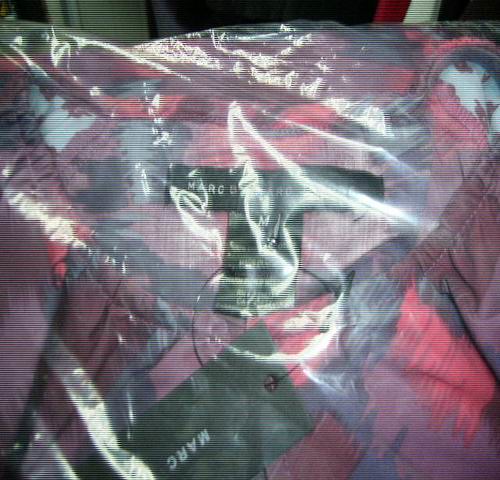The photograph depicts a brand new Marc Jacobs clothing item, still in its original, unopened plastic packaging. The garment, which looks like a dress, has a vibrant tie-dye and patchy color scheme featuring shades of pink, purple, red, and dark blue. The fabric appears to be adorned with a floral pattern that includes white and pink flowers. Visible through the clear plastic, the item bears a medium size label and a designer label; "Mario" can be partially seen, but a black tag with "Marc" in white letters is more distinct. Due to a glare on the plastic, possibly from camera flash, some details on the labels are difficult to read. The packaged dress is resting on a table, with its pristine condition and tags indicating it is brand new.